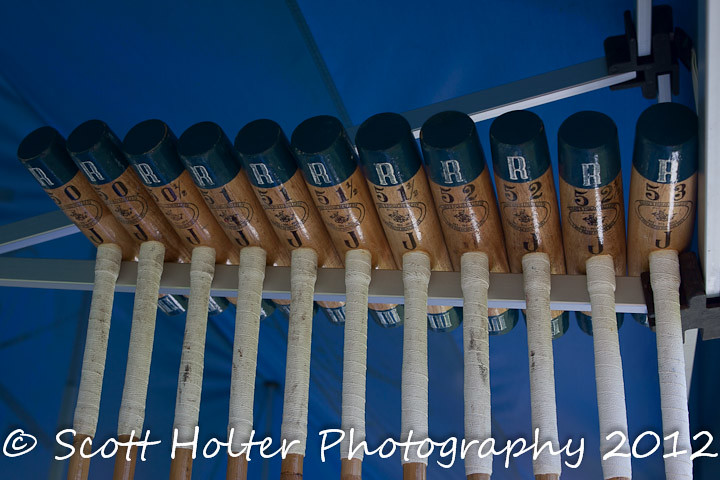The image captures an upward view inside a tent-covered structure featuring a blue ceiling. Prominently suspended from the ceiling is a sleek, silver metal holder which descends diagonally from the upper right to the lower left, forming a V-shape before extending horizontally. Attached to this metal framework is a series of brown wooden mallets, each distinguished by black ends. The mallets bear unique numbers - 50, 51, 52, and 53 - alongside silver Rs and black Js. The setup is visually striking against the overhead canvas or heavy plastic cover, creating an intriguing juxtaposition of materials and shapes. The bottom of the image is marked with the caption "Scott Holter Photography 2012," identifying the photographer and the year the photo was taken.